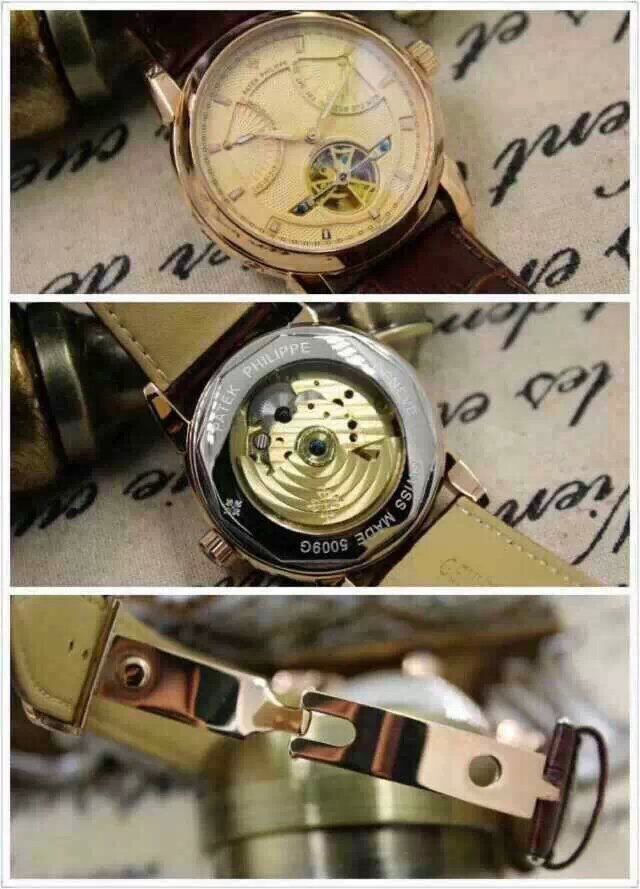A collage of three detailed photographs showcases an intricate wristwatch. The top image captures the complete watch: it features a white face adorned with a central gear reminiscent of a windmill, flanked by two semi-circular compass-like indicators at the top left and right corners. The watch is placed on a sheet of white paper bearing black text. The middle photograph reveals the watch with its face removed, revealing striking silver edges inscribed with fine writing and a golden metallic center. The watch band is a light tan shade, adding a touch of elegance. The bottom photo zooms in on the clasp, which has a polished copper, or possibly bronze, finish. In the background, a bronze ring encircles a cylindrical object, adding an extra layer of detail and texture to the composition.